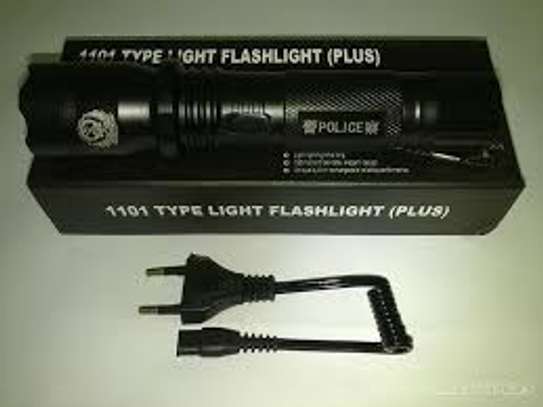The photograph features a black rechargeable flashlight prominently positioned on top of its box. The flashlight, roughly six inches in length, is labeled "police" on the handle and displays an insignia near the bulb. The box, also black, showcases the text "1101 type light flashlight" with "plus" in parentheses, printed in white across the top and edge. Below the box, a coiled charging cord is visible, designed to connect the flashlight to an electrical outlet for charging. The image is set against an off-white background with a greenish tone, possibly due to the lighting during the photo shoot. Additional small, unreadable text can be seen beneath the flashlight within the box.